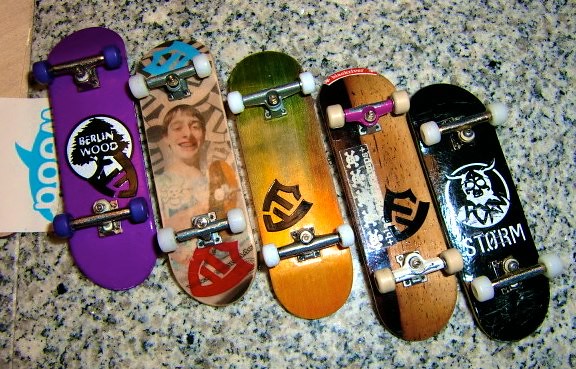This is a detailed photograph in landscape format showcasing five miniature skateboards, wheels facing up, arranged on what appears to be a granite countertop. From left to right, the first skateboard features blue wheels, a purple deck, and a black tree against a background that reads "Berlin Wood" in white letters. It also has a partial image of a shark. The second skateboard displays a photograph of a smiling young boy with braces accompanied by a red badge beneath the image. The middle skateboard has a gradient design, blending orange at the bottom into green at the top, and displays a black badge possibly inscribed with "FF". The fourth skateboard maintains a natural wood finish, equipped with cream wheels and bearing the same "FF" logo. The final skateboard on the right has white wheels and a black deck, adorned with a chalk-like drawing of a man with horns above the word "STORM" written in white letters. These intricate designs suggest that the skateboards might actually be fingerboards used for performing tricks with fingers rather than being full-sized boards.